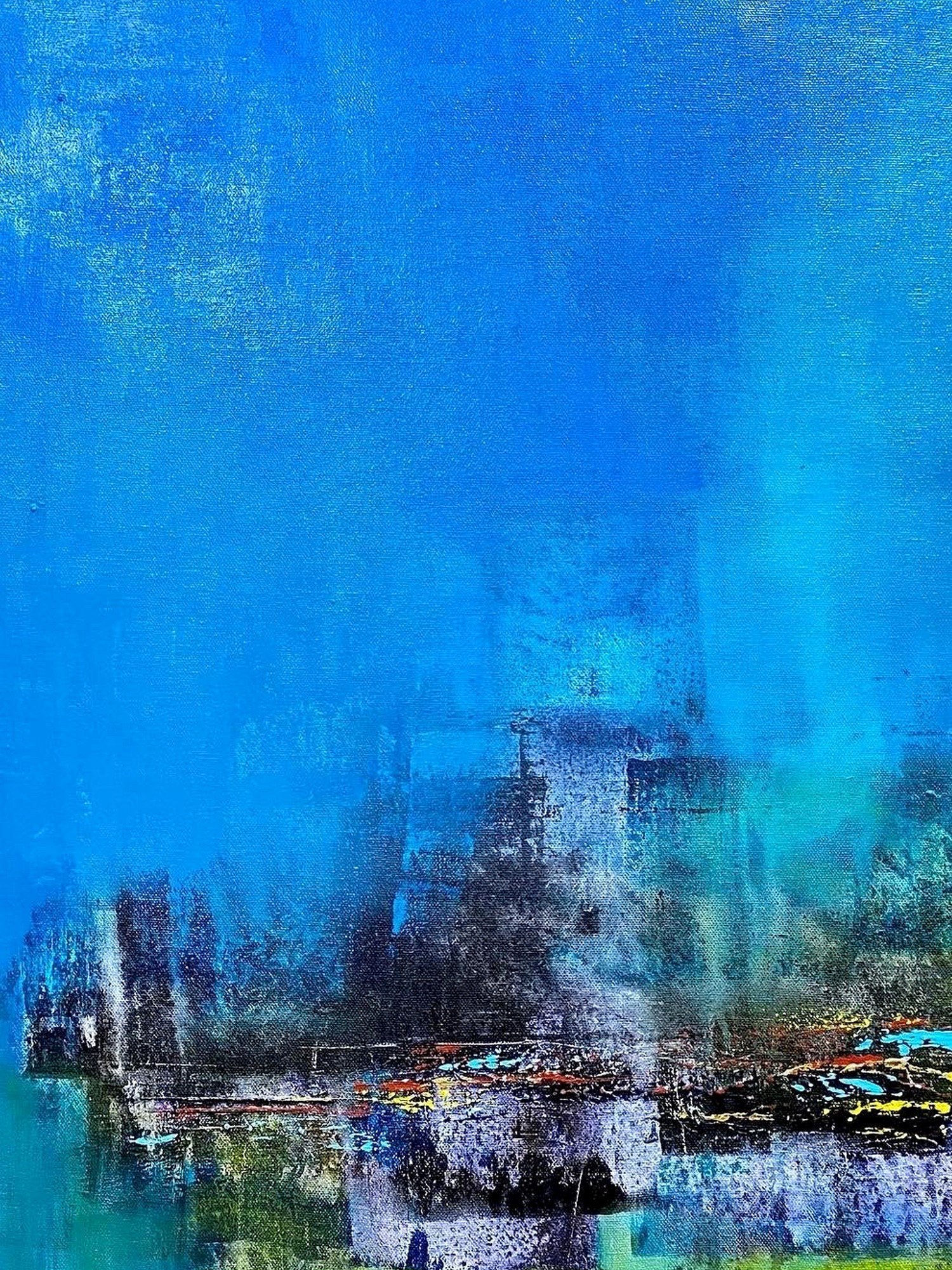This vertical rectangular painting features a two-toned blue background transitioning smoothly from a darker blue in the top left corner, dotted with hints of green, to increasingly lighter shades towards the middle and then down to the right-hand side. The upper portion predominantly showcases various hues of blue, punctuated by touches of black and green, giving the impression of a layered sky. Moving towards the middle of the painting, the colors darken, revealing a more complex scene that resembles an abstract structure or the side of a building, with a white front and a possible black window-like feature. Below this midpoint, the image grows more intricate, portraying a chaotic mix of colors such as purple, yellow, red, and light blue. These colors appear splattered and spray-painted, creating a vivid and somewhat distorted lower half that suggests either a reflection in water or a blurred landscape. Vertical white strips in the bottom right corner add to the ambiguity, possibly hinting at water or cascading elements. The entire composition is intricate and somewhat abstract, with elements that hint at urban decay, natural reflections, or even floral imagery, albeit in a hard-to-decipher style that leaves much open to interpretation.